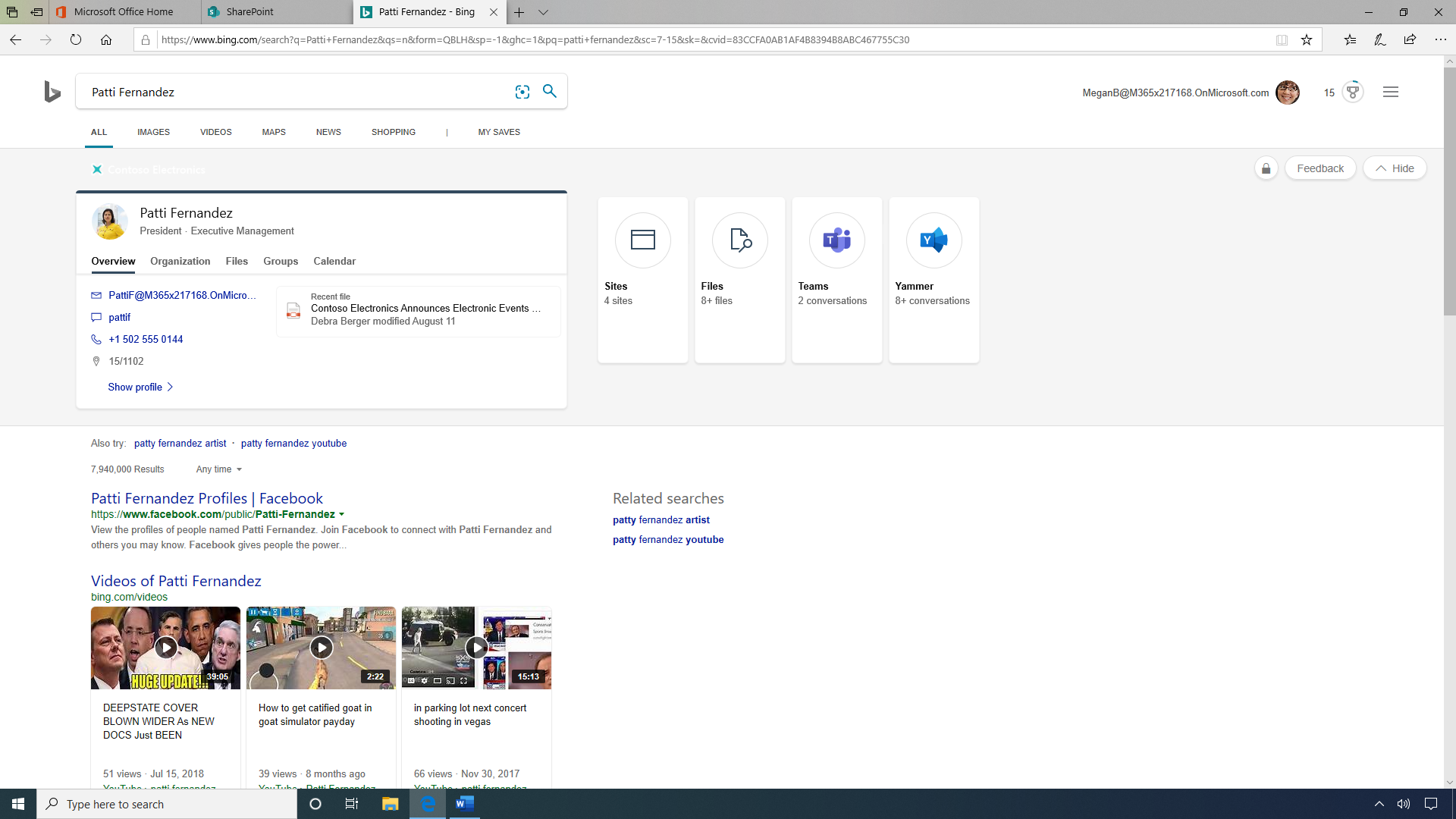In this image captured from a Bing search page, the interface is laid out cleanly on a white background. At the top, the Bing search bar prominently features the query "Party Fernandez," accompanied by a distinctive "B" icon signifying the Bing search engine. Below the search bar, a variety of navigation tabs are available: All, Images, Videos, Maps, News, Shopping, and My Saves.

On the top right corner, a user identified as MeganBee (MeganBee@M365X217168.onMicrosoft.com) is logged in, with a Bing Points tally of 15. Directly beneath the search bar, there is a highlighted profile summary for Party Fernandez, identified as President, Executive Management. This section includes tabs for Overview, Organization, Files, Groups, and Calendar, with all text appearing in black except for an email address (PartyF@M365X217168.onMicrosoft.com), which is in blue. Additionally, a contact number "+1 (502) 555-0144" is listed. The profile location is specified as "05-1102," with an option to "Show Profile."

To the right of the search results, the "Recent Files" section references a file titled "Contacts for Electronic Announcements" by Debra Pekka, modified on August 11. Below, suggestions prompt further searches, including "Party Fernandez Artist," "Party Fernandez YouTube," and a context note stating there are 7 million and 40,000 results anytime.

Under "Also Try," a search result is listed with the title "Party Fernandez Profile" on Facebook (URL: facebook.com), inviting users to view profiles and connect on the platform. Another result highlights "Videos of Party Fernandez," hosting three specific videos: "Deep State Carver, Blown Wide as New Docs Just Been," "How to Get Clarified Codes in Code Simulator Payday," and "In Sparking Lot, Next Content Shooting in Vecas." Titles are in blue, while URLs are displayed in green.

The cumulative visual content includes four dedicated sections for Files, Teams, Yammer, and Conversations, indicating interactive elements and collaborative features.